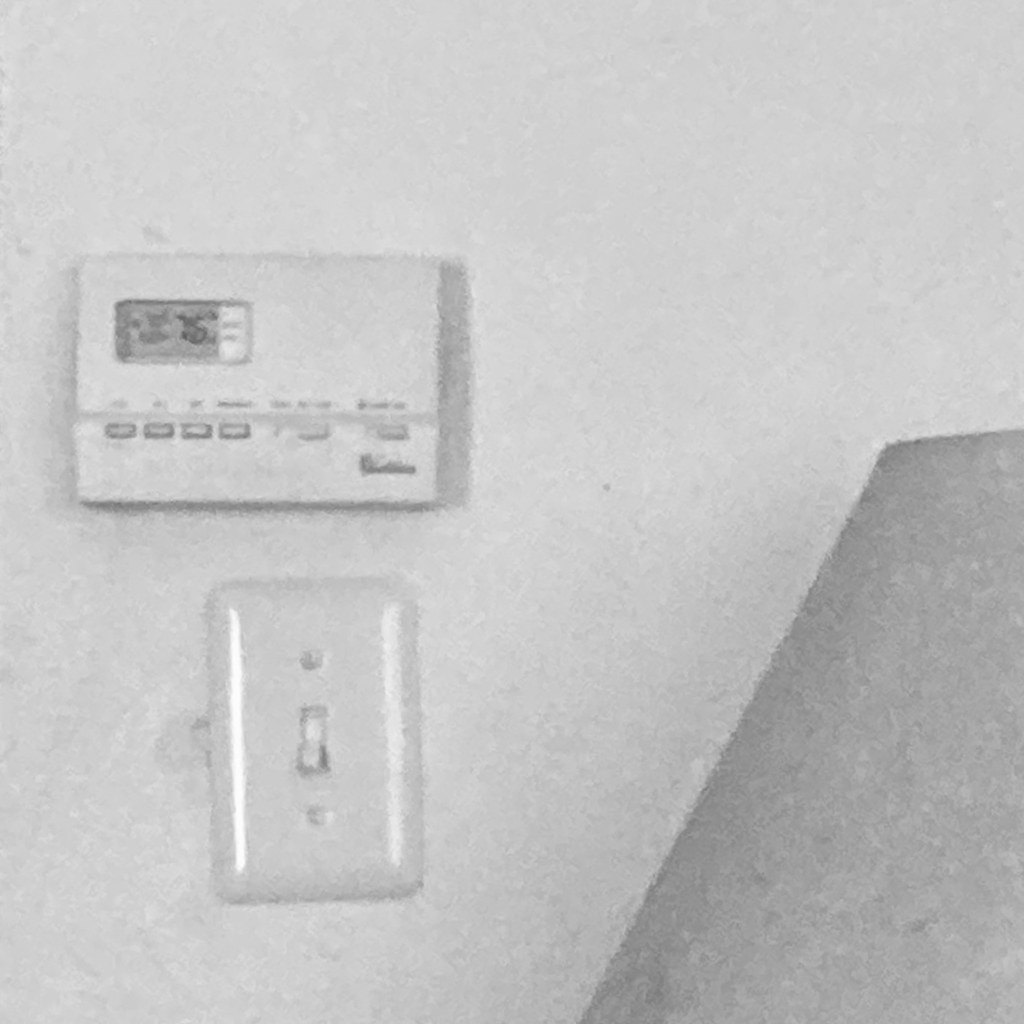A grainy, nearly black-and-white photograph captures a white wall featuring several items. A white light switch with its toggle in the down position and a matching white faceplate is situated prominently. Above the light switch, a white thermostat is mounted. The thermostat, showing a temperature of 76 on its LED screen, has four buttons beneath the display and two additional buttons to the right. Text, presumably the manufacturer's name or model information, is located on the corner of the thermostat unit. An unidentified object, possibly resembling a shelf, extends diagonally across the bottom right section of the image, not aligning parallel to either the thermostat or the light switch. The stark white tones of the wall and devices, coupled with the poor image quality, give the impression of an almost monochromatic scene.